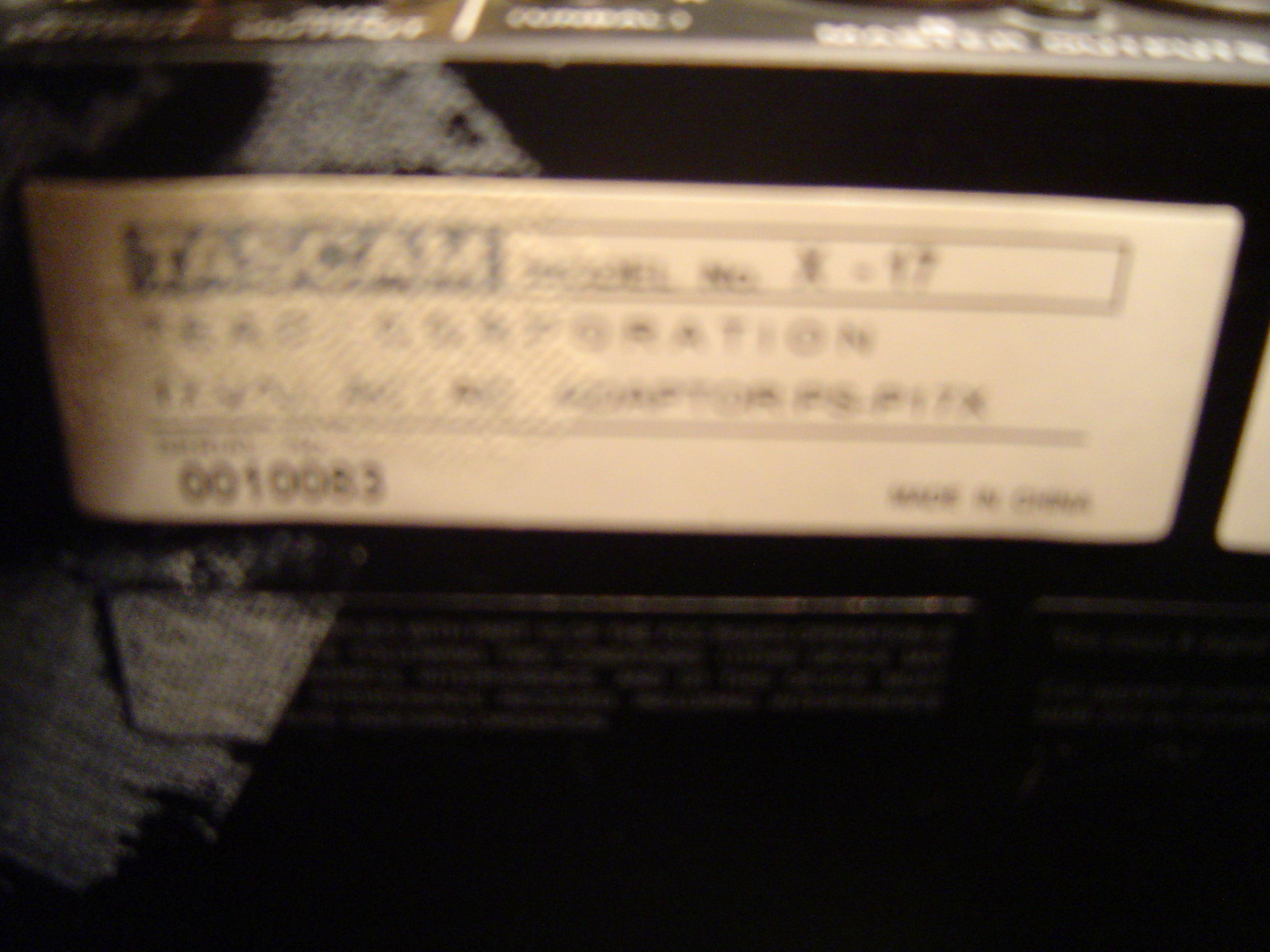This is a very close-up, blurry image of a label on a rectangular black object, likely made of plastic or metal. The label, which seems to be a sticker, is predominantly white with a faint black border and is somewhat stained and dirty. The main focal point is the brand name 'TASCAM' printed in blue and white, located at the top left of the label. Below the brand name, there is more text, possibly detailing the model number and other specifications, but it is illegible due to the blurriness and dirt. Additionally, in the bottom left corner of the label, there is a series of numbers that appears to be '0010003' or similar. In the bottom right corner, the words 'Made in' are faintly visible, but the location is unclear. The bottom of the label contains more text that seems to be some type of regulation or warning information, but it is too blurry to decipher. Despite the difficulty in making out all the details, the label indicates that the object is likely a piece of camera or sound equipment.